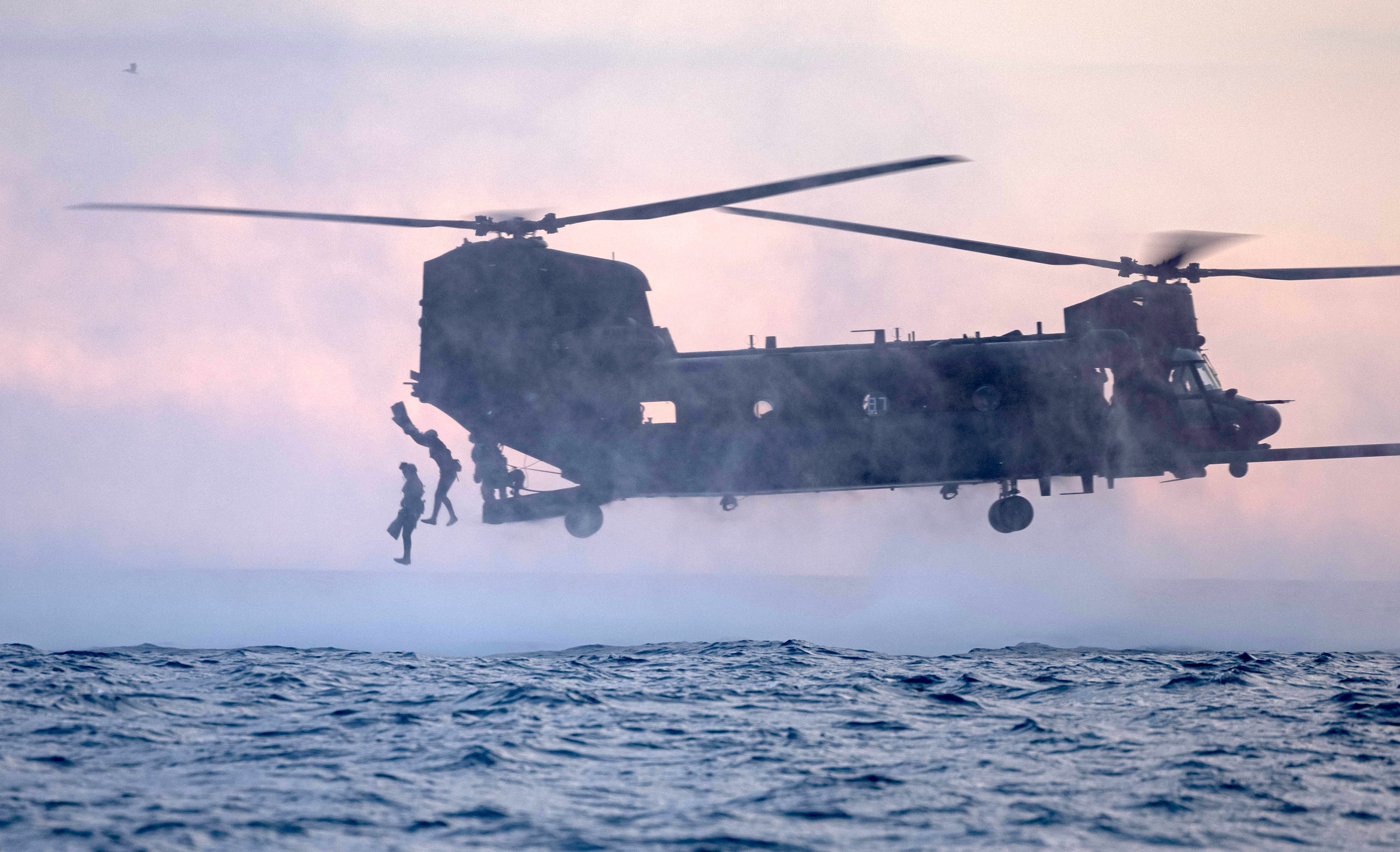In this dramatic photograph, a large, black helicopter, potentially a military Chinook, hovers above rippling ocean water with a striking pink and blue skyline in the background. The imposing aircraft, with its elongated body and two massive propellers, appears to be engaged in a military operation. Dark silhouettes of soldiers are visible, some mid-air as they leap from the rear ramp into the water below. The propellers blur with motion, enhancing the sense of urgency and activity in this powerful scene. Scattered details like the undercarriage wheels and side windows provide a faint glimpse into the helicopter's structure, while the sky's gradient colors highlight the stark contrast between the mechanical craft and the natural evening backdrop.